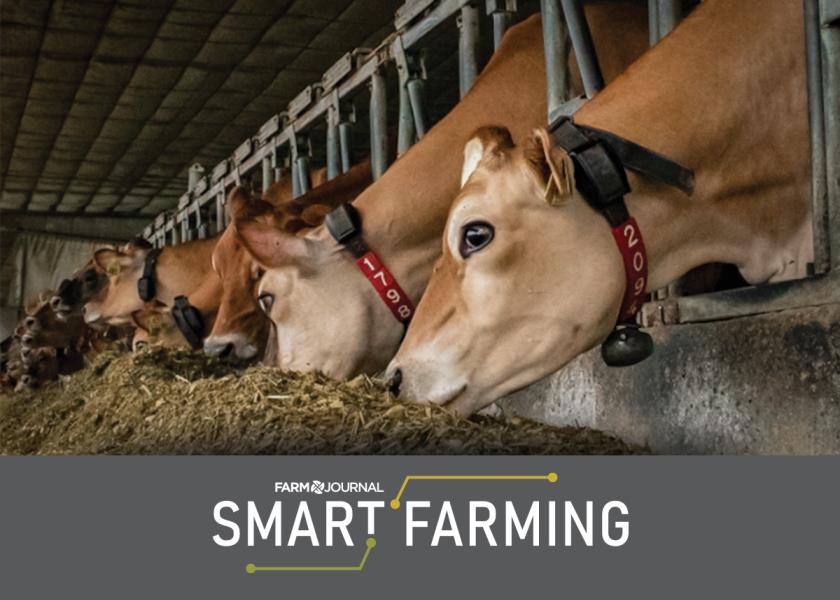The image depicts a farming environment within a spacious barn facility featuring a row of cows standing in their pen, each with its head extended through a gate to feed on hay. Noticeably, every cow is equipped with a collar that includes various technological components such as a battery box and an electronic device, likely for monitoring purposes. The collars are uniquely numbered with four-digit identifiers, ensuring each cow can be easily tracked. Prominently displayed within the photo is a gray band with white text that reads "Farm Journal Smart Farming," indicating the integration of digital technology in modern farming practices.